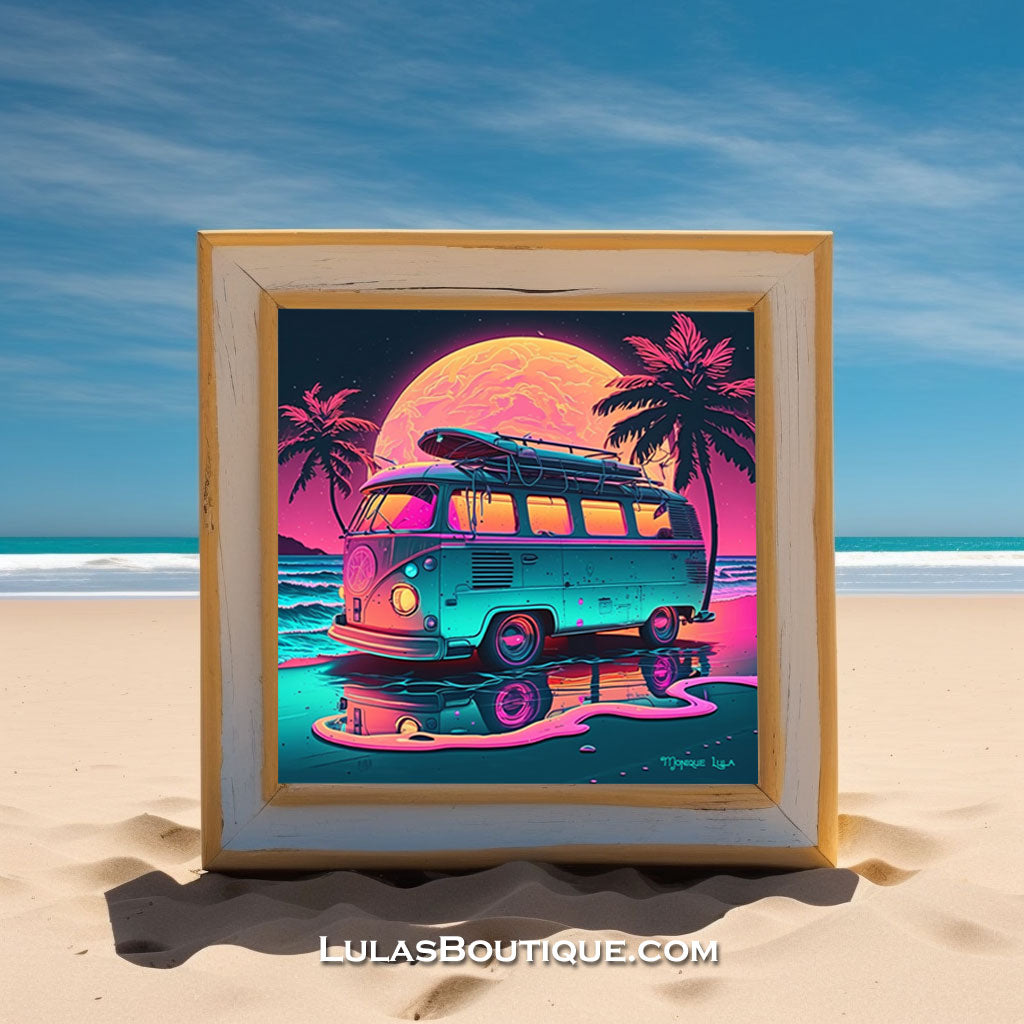The image portrays a serene beach scene with a pale light beige, smooth sand at the bottom, a light turquoise ocean with gentle foamy white waves in the middle, and a clear blue sky with faint white clouds at the top. Centrally placed in the foreground is a standout square picture frame, accented by a yellow and white border. Inside the frame is a vibrant neon-colored depiction of a retro teal Volkswagen microbus, adorned with a surfboard on top. This microbus, reflected in the water it's parked on, is set against a beachscape under a magenta and cyan color scheme reminiscent of the 80s. Flanked by two palm trees, one behind and one seemingly emerging from the passenger side, the scene features a great big ball behind the bus, interpreted as either the sun or the moon. The bottom of the framed picture bears the artist's name and the website “lulasboutique.com.”